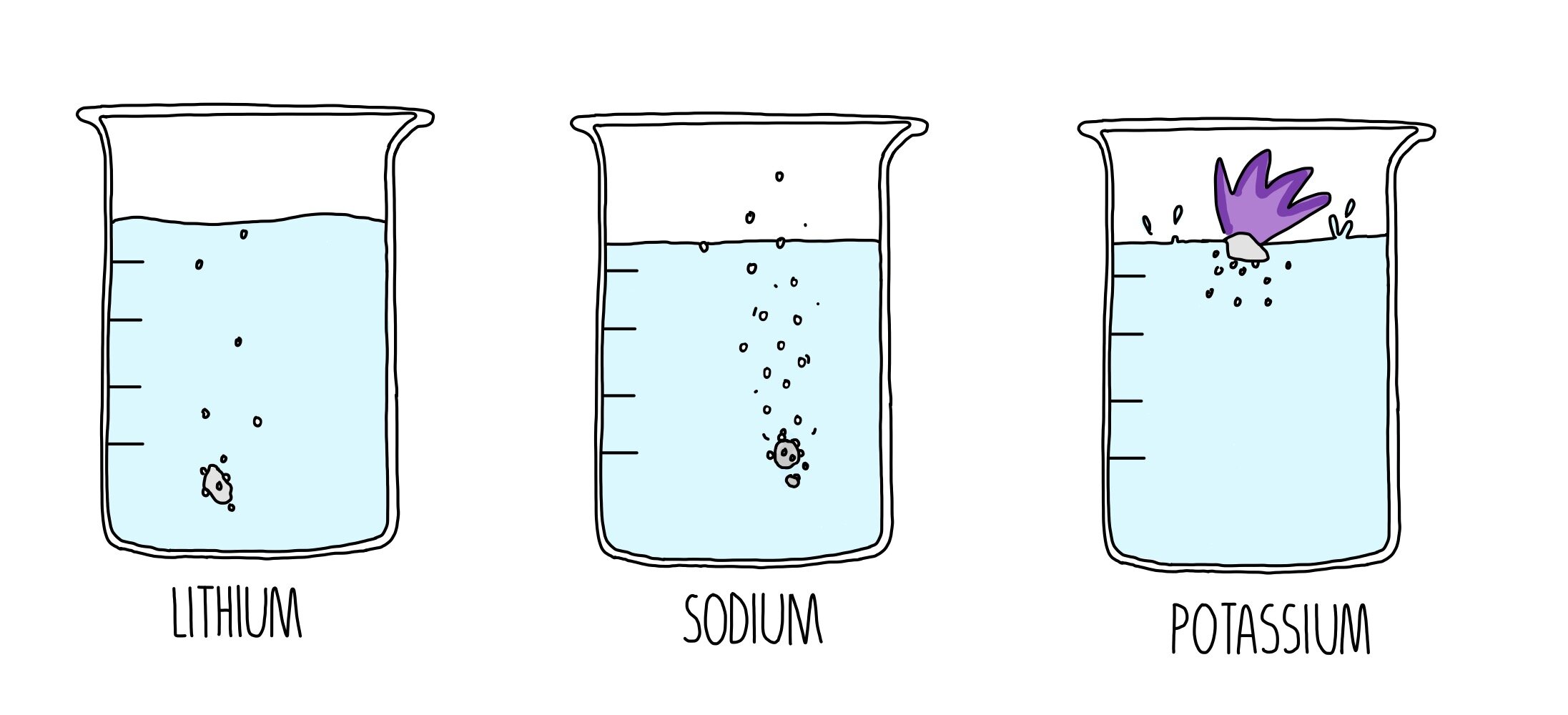This illustration is a cartoonish and clip-art style diagram of three glass beakers, all outlined in black with measurement markings along their sides, set against a plain white background. Each beaker is filled with a pale, light blue liquid up to a wavy black line. Underneath each beaker, there are clear labels in black capital letters: Lithium, Sodium, and Potassium, respectively. 

In the first beaker labeled "Lithium," there is a gray pebble sinking at the bottom, accompanied by a few small bubbles rising to the surface. The second beaker, labeled "Sodium," shows a larger pebble near the bottom with numerous bubbles spreading upwards, even extending above the liquid level into the white space of the beaker. The final beaker, labeled "Potassium," features a rock-like piece floating near the surface, with smaller particles drifting downwards. Additionally, a purple explosive shape with water droplets splashing out from the top is prominently featured, symbolizing a more vigorous reaction.